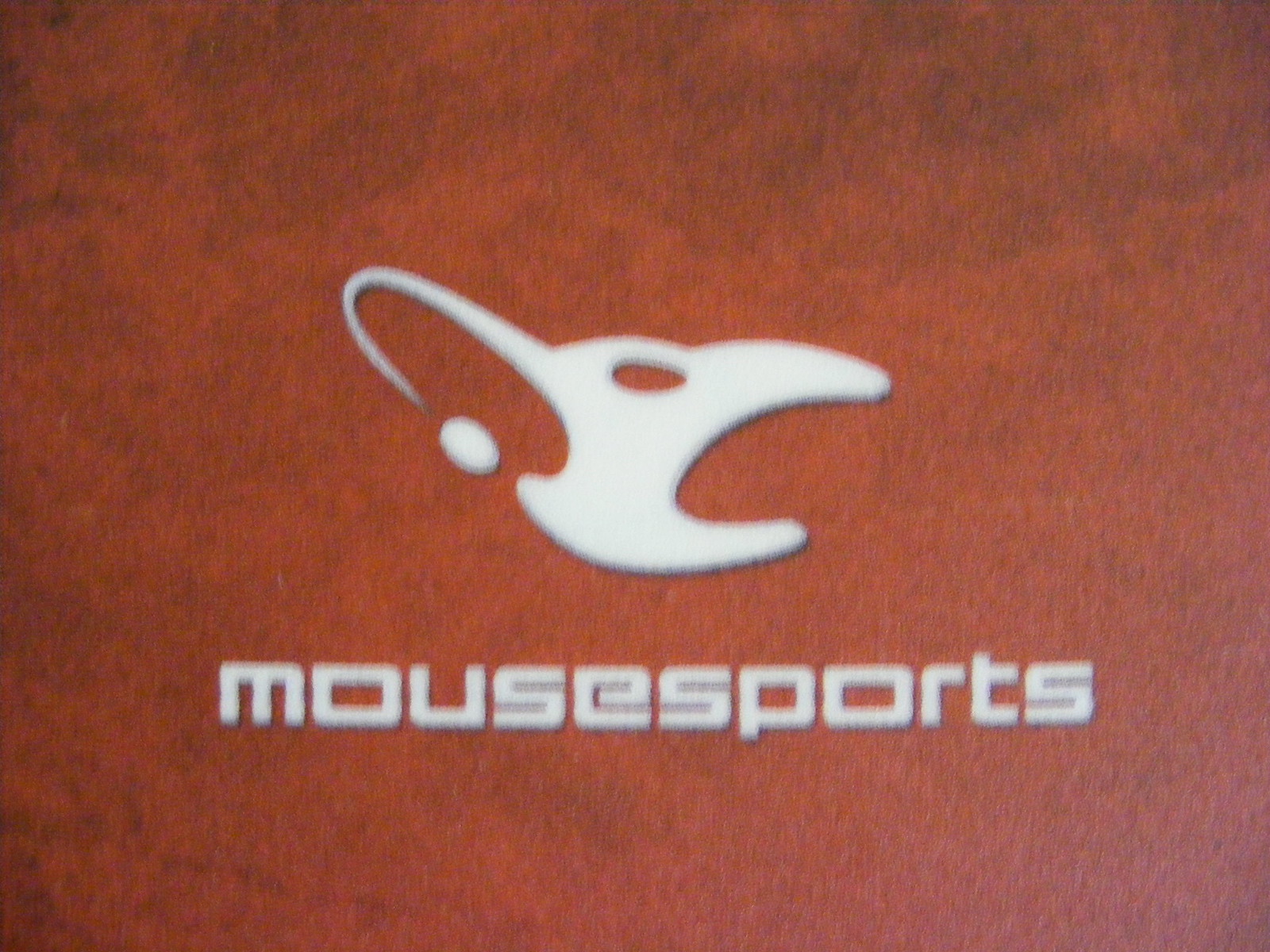This is a close-up image of a modern, stylized logo imprinted on a textured leather surface, which is predominantly brown with black smudges for added depth. The logo itself is a highly simplified and stylized representation of a mouse head in white, viewed from its right profile. The mouse features a cut-out oval for an eye, an open mouth, and a lozenge-shaped line for an ear that terminates in another white oval. This creates a striking image using negative space. Below the mouse logo, in all capital letters and modern blocky sans-serif font, the text "MOUSE SPORTS" is prominently displayed. The overall design, with its mix of futuristic typography and minimalist iconography, makes for an eye-catching visual against the darkened leather background.